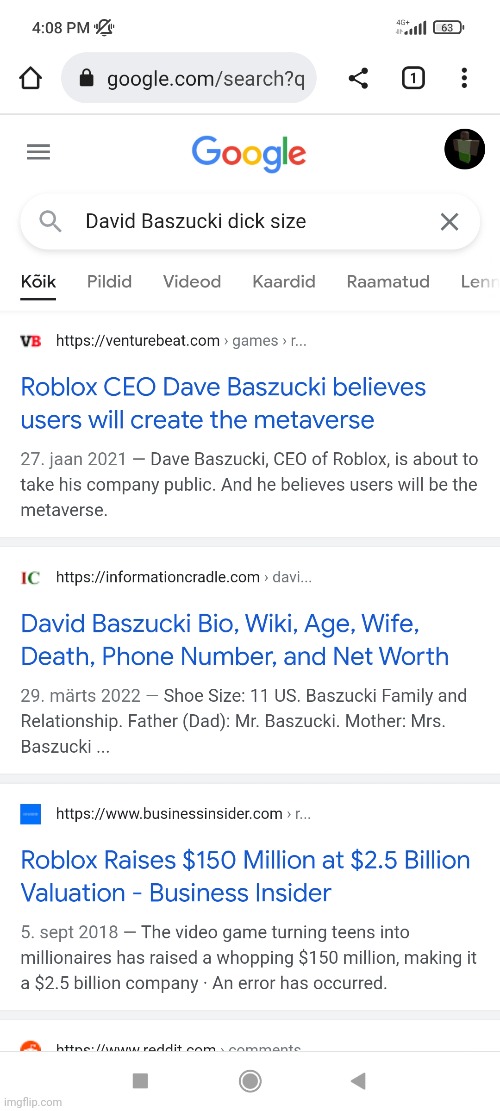This is a detailed descriptive caption for an image:

The image is a screenshot of a Google mobile search interface. The background is predominantly white, with the iconic Google logo displayed at the very top center. Just below the logo, within the search bar, the query "David Bazooki dick size" is typed out. Directly beneath this search bar, the initial search result appears, featuring a headline that reads, "Roblox CEO Dave Bazooki believes users will create the metaverse," misidentifying the inquiry about the Roblox CEO's genital size. 

A user profile photo, enclosed in a circular frame, is visible at the top-right corner of the screen, indicating the active user. At the screen's bottom center, standard mobile navigation icons are present: a home or minimize icon in the middle, a right-facing arrow on the left, and a square on the right. Additionally, at the very bottom-left corner of the screen, there is a small, slightly faint watermark that reads "imgflip.com."